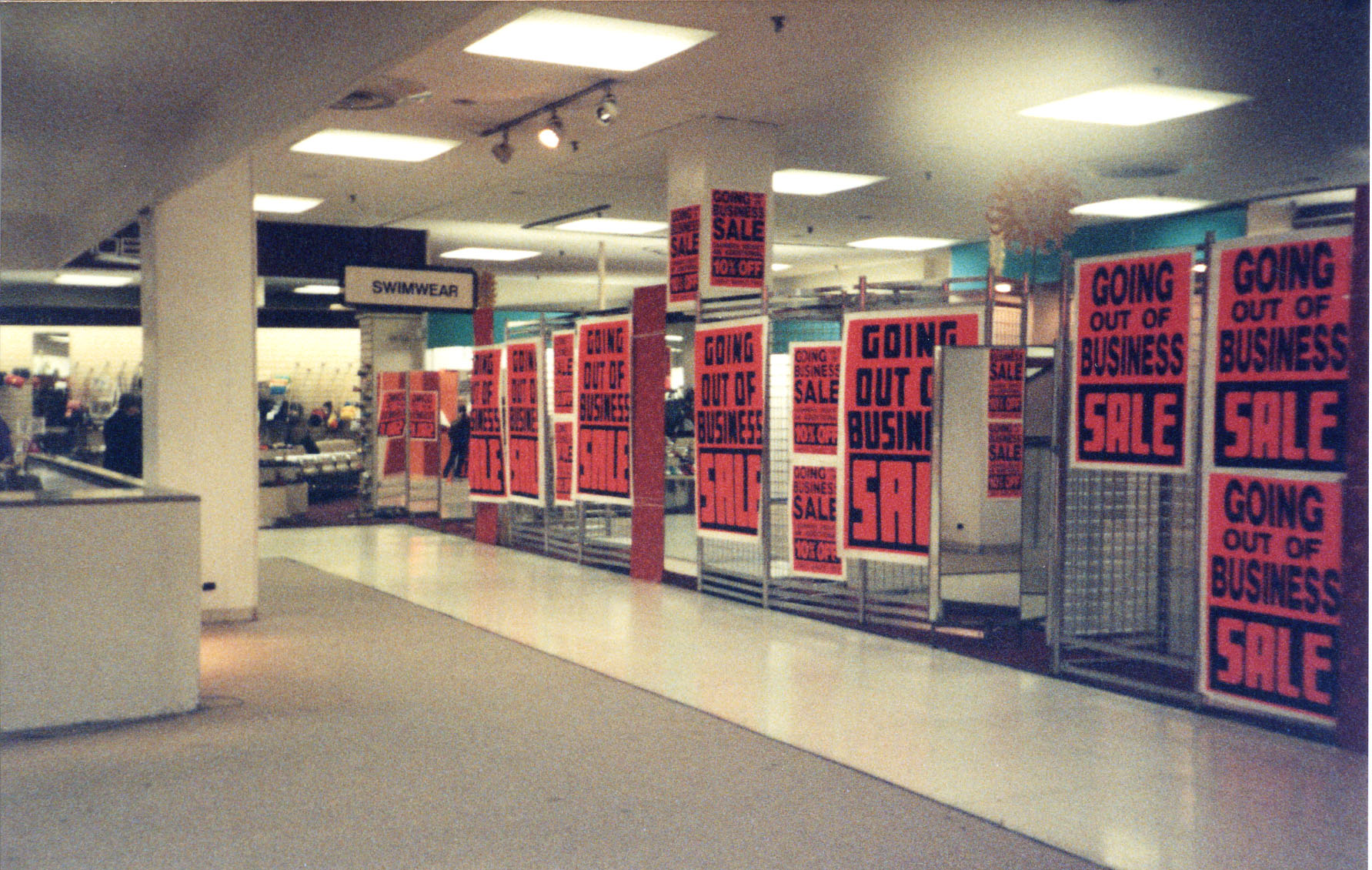Inside the image, there appears to be the interior of an old-fashioned department store, likely photographed around 20 years ago. The store is in the midst of a "going out of business" sale, evident from the numerous orange signs with white borders and black text announcing the sale. Approximately 15 or more of these signs are prominently displayed on various racks on the right side of the image. 

On the left side of the image, there is a small table that could be used for customer service purposes, next to a white pillar. Near the ceiling in the background, a sign indicates the location of swimwear. The ceiling itself features several lights, providing ample illumination to the space. Further back, there appears to be an area designated for handbags or similar items. 

The flooring varies in different parts of the store; the majority appears to be white tile, while the left-hand side includes a section covered in carpet, adding to the dated ambiance of the store layout. The overall scene captures the atmosphere of a once-bustling retail space now in the throes of winding down operations.